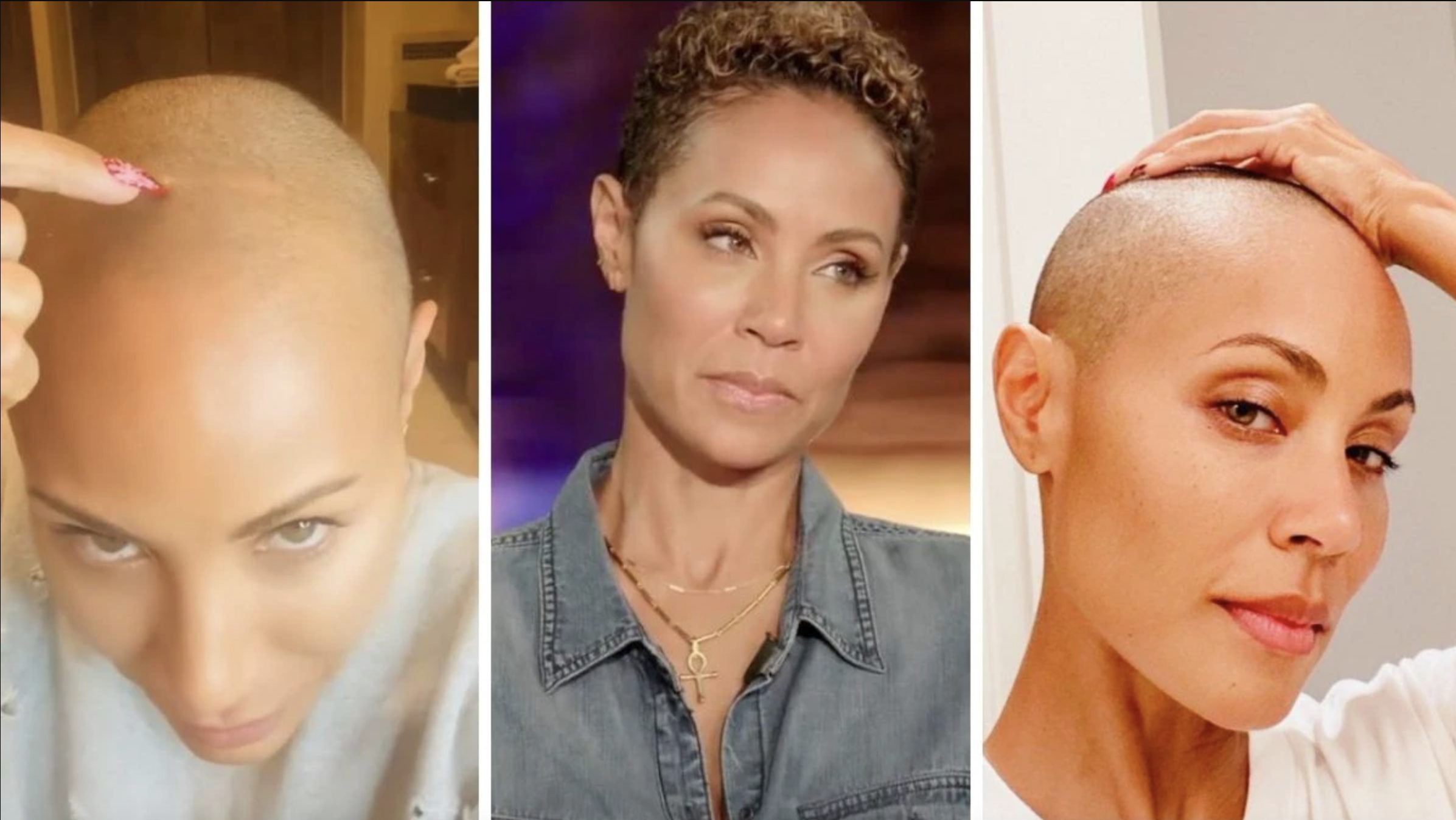This triptych image showcases three separate vertical photographs of actress Jada Pinkett-Smith, each partitioned by a thin white border. In the leftmost photograph, Jada is bald and pointing to a specific spot on her head with her red-painted fingernail, slightly lowering her head. She is attired in a white shirt, and the background depicts a room with brown furniture and cream-colored walls. The middle photograph presents Jada with very short, curly, brown hair, slightly tilting her head towards the right. She is adorned in a denim-like blue jacket and two gold necklaces, one featuring a cross. The backdrop includes a mix of purple, brown, and tan hues. The rightmost image shows a bald Jada once more, with her left hand resting on top of her head. Her eyebrows are precisely manicured, and she gazes at the viewer with a model-esque pose. She wears a white shirt, and the background consists of white walls with a potential hint of a window on the left side. Overall, the detailed elements in each photograph highlight Jada's expressions, attire, and the distinct backgrounds seamlessly capturing different moments and moods of the actress.